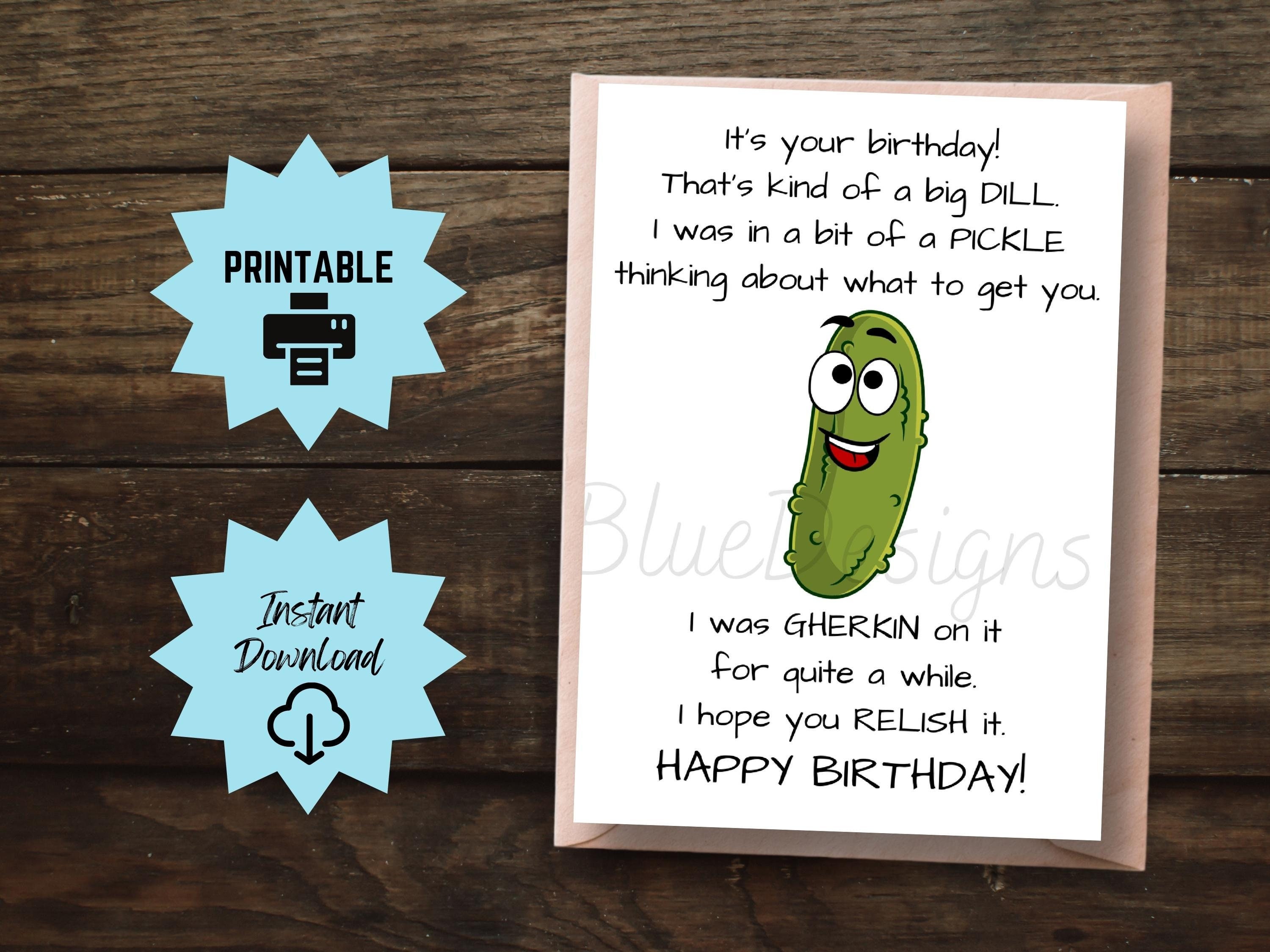The image is an online advertisement for a humorous birthday card, set against the background of a wooden surface displaying the texture and grooves of wooden boards, sprinkled with a few crumbs. On the left of the image are two blue starburst-shaped icons. The top one reads "PRINTABLE" in bold, black, all-caps text with an adjacent printer icon, while the bottom one reads "Instant Download" in mixed-case marker font, accompanied by a cloud and download arrow icon.

The centerpiece is the birthday card itself, which features a white card with a pink outline, showcasing a cartoonish, smiling pickle with eyes. The card humorously states, "It's your birthday. That's kind of a BIG DEAL. I was in a bit of a PICKLE thinking about what to get you. I was GHERKIN on it for quite a while. I hope you RELISH it. HAPPY BIRTHDAY," with certain words emphasized in all caps. The creator's watermark, "Blue Designs," is subtly overlaid on the pickle. The overall composition is both cute and humorous, designed to bring a smile to the recipient's face.